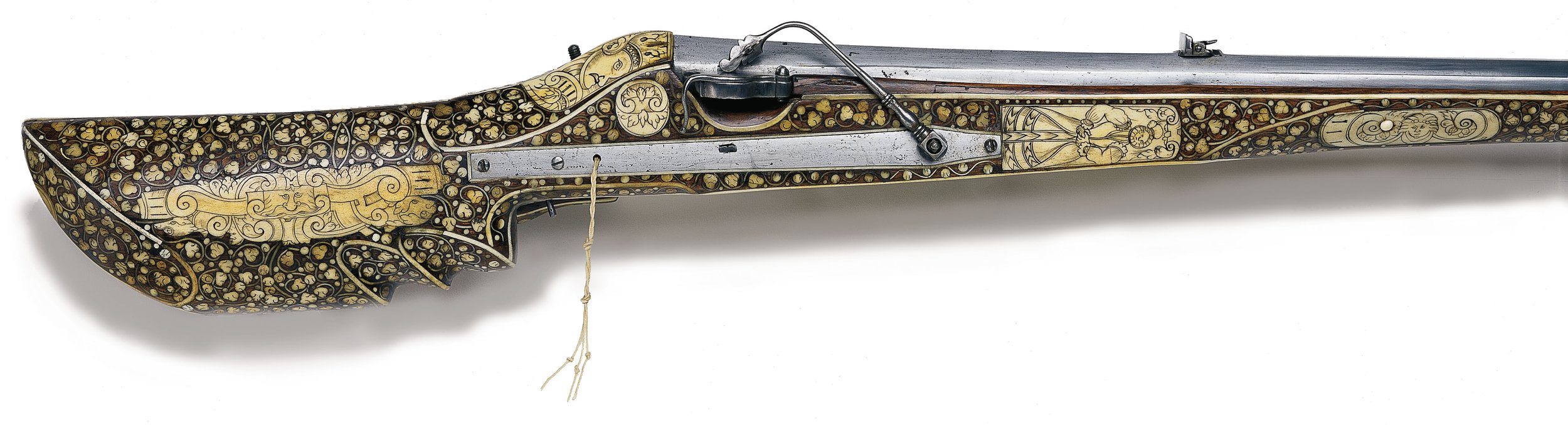The image depicts a decorative weapon with a complex design set against a white background. The central object appears to be a flintlock pistol, though it also incorporates elements that might suggest a rifle or another kind of historical weapon. Intricate details include a serrated blade-like top portion, and the whole piece is adorned with an ornamental, almost mythological style that suggests it could be a sheath or part of an elaborately designed tool.

The handle and body feature a golden-black texture with smooth surfaces. Silver accents are present across the top and along the sides, prominently including the barrel, which is a defining characteristic. Artistry is evident with inlaid patterns and a variety of engravings: faces, potential knight figures resembling medieval times, along with small, pale mushroom-like motifs. Distinctly, the knight depiction and drawn heads in black, brown, and tan add to the medieval, ornamental appeal.

Notable features include a prominent golden emblem at the handle and trigger area, which emphasizes its decorative nature. There's a thin piece of rope hanging through a small hole near the bottom, suggesting functional detail or further decoration. Along the barrel, two golden labels display images, one of a horizontal man and another with a cloud-like figure, enhancing the mythological and intricate design of the piece.